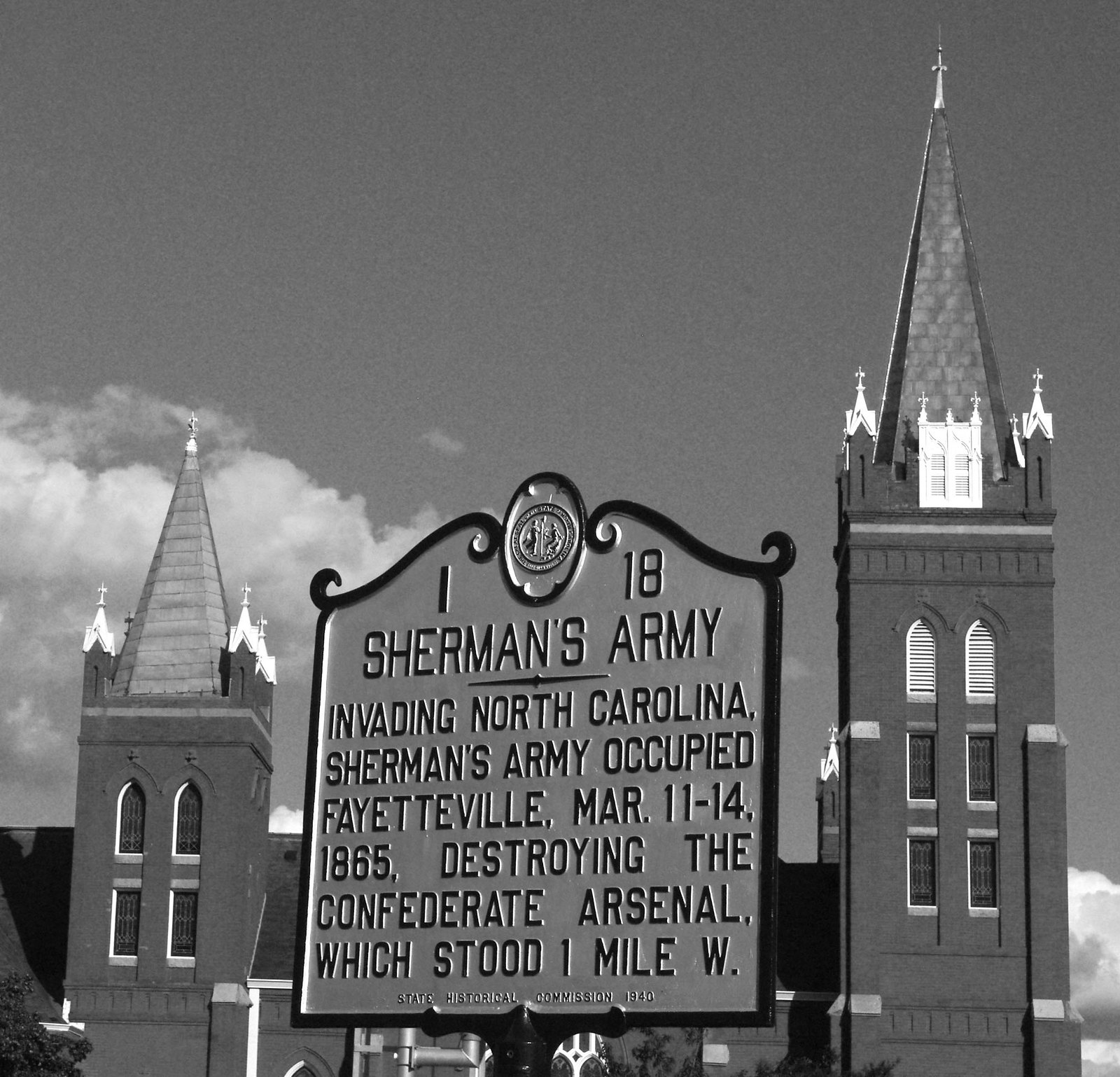This black-and-white photograph, characterized by its over-saturated grayscale tones, captures a historical marker positioned in front of a church. The church features two prominent steeples with arched windows; notably, the steeple on the right is taller than the one on the left. The sky, occupying the top two-thirds of the image, is marked by whitish-gray clouds, providing a stark contrast to the dark, detailed silhouette of the building.

The historical marker at the center of the photograph bears inscriptions in raised, light-colored print. At the top-left corner is a "1" and at the top-right is an "18". Beneath this, in uppercase letters, it reads "SHERMAN'S ARMY", followed by a horizontal separator. The main text of the marker states, "INVADING NORTH CAROLINA. SHERMAN'S ARMY OCCUPIED FAYETTEVILLE, MARCH 11-14, 1865, DESTROYING THE CONFEDERATE ARSENAL, WHICH STOOD ONE MILE WEST." At the bottom, the marker notes, in smaller print, "State Historical Commission 1940." The scene highlights a significant historical reference amidst the serene yet somber backdrop of the old church and cloudy sky.